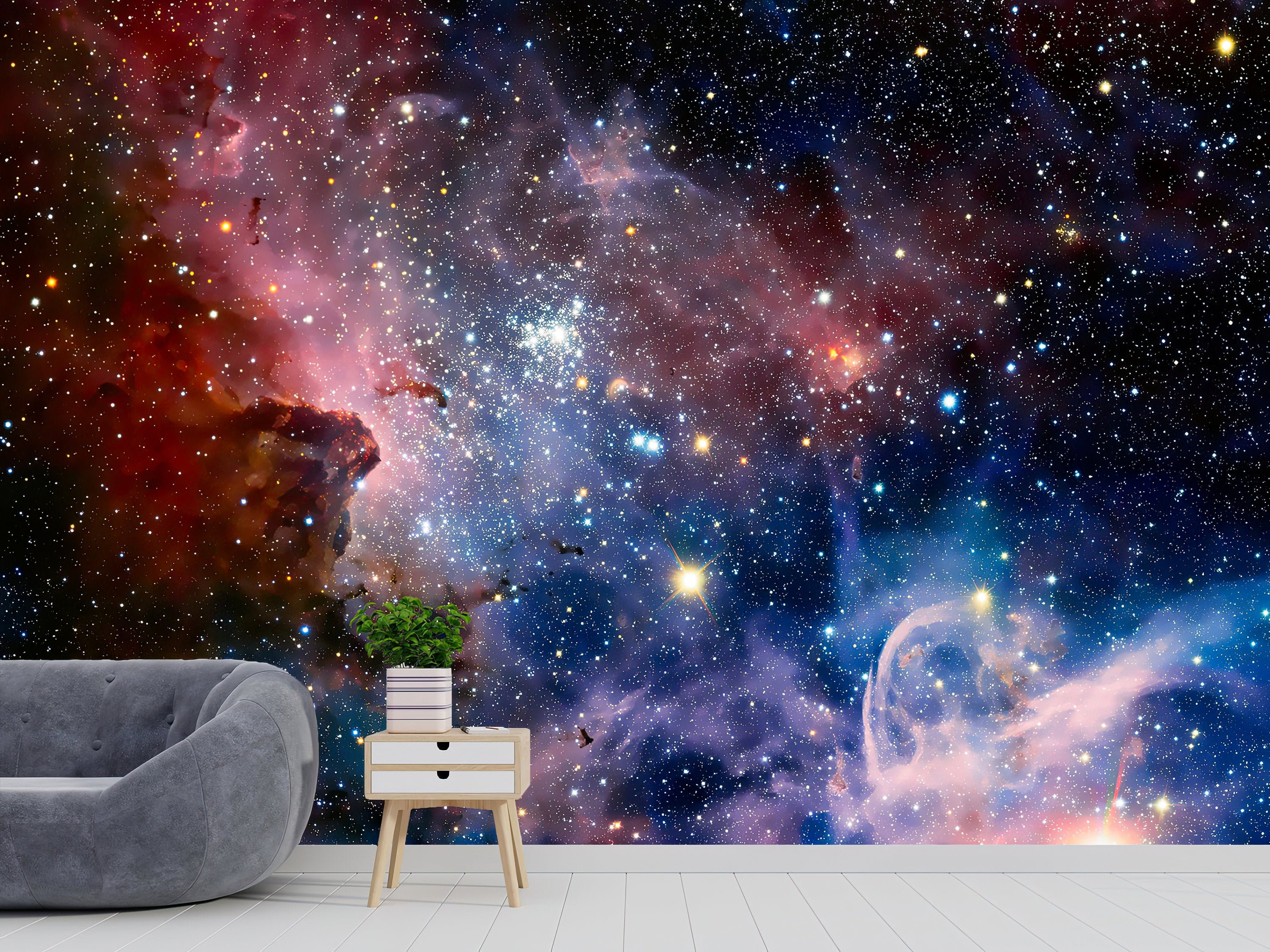The image depicts a room with a striking galaxy-themed wallpaper that spans the entire wall behind a modern gray couch, positioned on the bottom left. The wallpaper vividly illustrates a star-studded cosmos filled with countless bright dots symbolizing stars in shades of red, yellow, white, and blue. On the left side of the wallpaper, there are distinct red gaseous clouds, likely depicting remnants of stellar explosions or other cosmic phenomena. Moving across to the right, the mural transitions to shades of blue and pink with a darker, almost black sky backdrop on the upper right.

In front of this galactic mural, the sleek gray couch adds a modern touch to the room. Adjacent to the couch is a small end table made from light-colored wood, featuring two white drawers. Positioned on this table is a notebook and a small blue and white striped pot holding a green plant. The room’s flooring consists of white wood, contributing to the contemporary and clean aesthetic of the space. The overall setting combines the wonders of the universe with modern interior design, creating a space that is both intriguing and stylish.